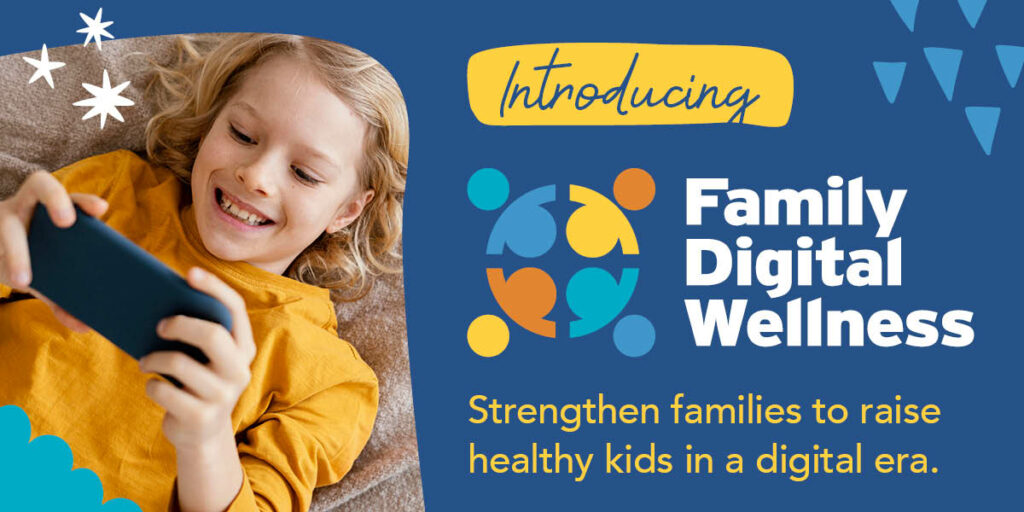This vibrant advertisement features a charming photograph of a young girl, estimated to be around 10-12 years old, with blonde hair, smiling as she looks at a blue cell phone she's holding sideways. She is dressed in a mustard yellow shirt and lies comfortably on a brown blanket. Above her hand-drawn white stars embellish the image. The right side of the ad transitions into a blue background, showcasing the text "Introducing Digital Family Wellness" written in white. Below, it continues with "Strengthen Families to Raise Healthy Kids in a Digital Era" in varying colors. Minimalist icons resembling family members holding hands and a series of small blue triangles adorn this section, adding to the overall playful and vivid design. The poster, marked mainly in blue, aims to promote healthy digital habits within families.